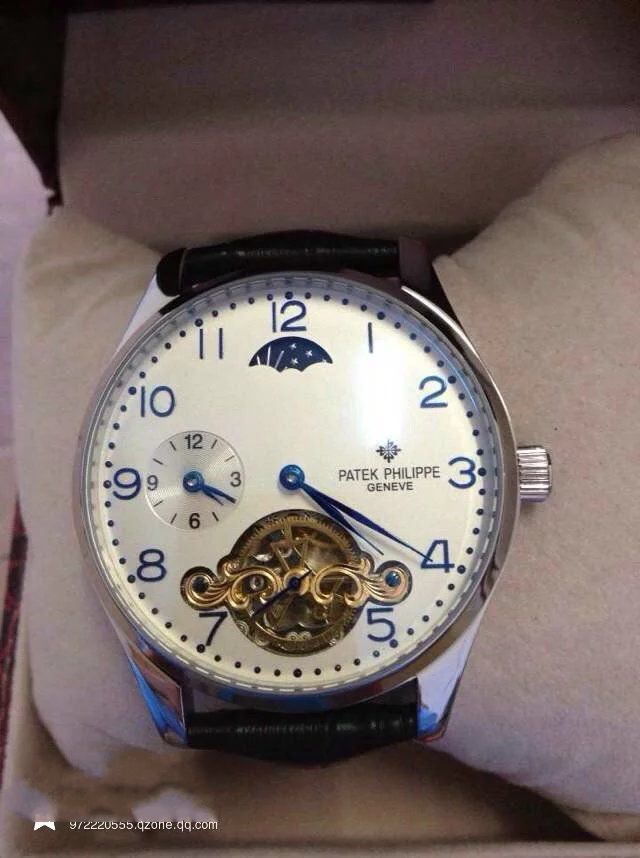The image displays a close-up of an expensive Patek Philippe watch, nestled inside its watch box. The black leather band of the watch is elegantly wrapped around a white cushion, as often seen with high-quality timepieces. The watch features a silvertone bezel with a cream face, adorned with large blue numerals at 12, 3, 6, and 9 positions, interspersed with smaller indicator dots. Additional smaller dials are present; one steampunk-style with visible mechanical elements and another modern-style dial, both contributing to the watch's sophisticated and intricate design. The primary hands of the main dial are blue, set to approximately 4:20. A web address "9-2-2-2-0-5-5-5.qzone.qq.com" is visible in the bottom left corner, possibly indicating the image's source. The brand "Patek Philippe Geneve" is prominently displayed next to the number 3, underscoring the watch's luxury and prestige.